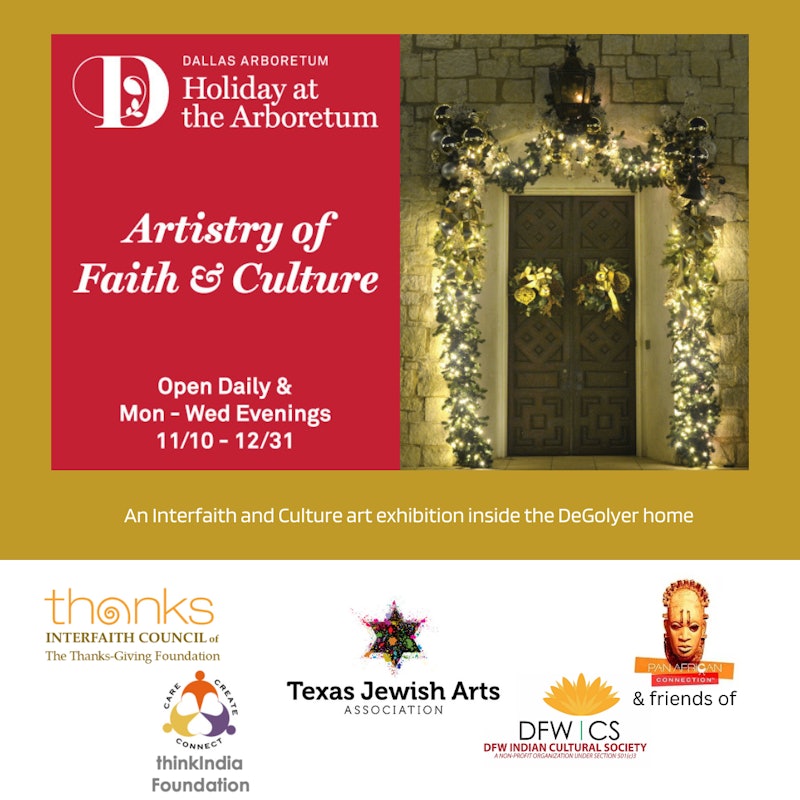This advertisement poster for the "Holiday at the Arboretum" event at the Dallas Arboretum features a visually striking gold background with a photo overlay. Dominating the left side is a prominent red square with white text that reads, "Dallas Arboretum Holiday at the Arboretum," followed by "Artistry of Faith and Culture." It also indicates the event's schedule, stating, "Open daily and Monday through Wednesday evenings, 11/10 to 12/31."

The right side of the poster showcases a captivating photo of a front door adorned with festive holiday decor. The doorway is framed with decorative, lit garland and features two wreaths, creating a Christmassy ambiance. A black lantern hangs above the door on a stone wall, enhancing the holiday spirit.

At the bottom of the poster, a gold trim features logos of various sponsors, including the Interfaith Council of the Thanksgiving Foundation, Texas Jewish Arts Association, Think India Foundation, DFW Indian Cultural Society, and Friends of Pan-African Connection. Additionally, the poster highlights that the event includes an interfaith and culture art exhibition inside the DeGoyer Home.